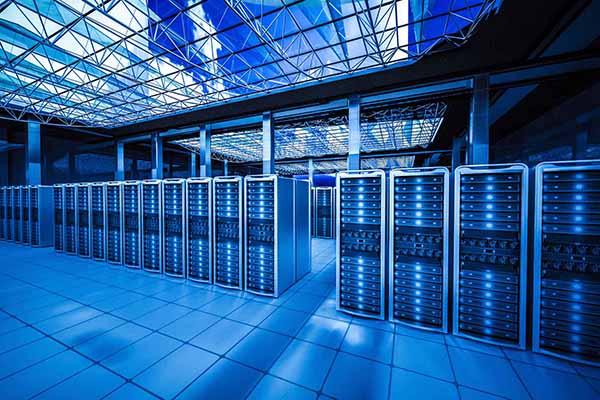This is an image, possibly a realistic digital artwork, depicting a pristine, industrial clean room with a monochromatic blue, white, and black palette. The spacious room features a tiled floor, meticulously clean, with rows upon rows of towering server racks or computer processing units, each as tall as a man. There are at least 30 visible towers, each split into six sections on both the top and bottom, with a blue light on every section indicating active operation. Overhead, the ceiling is composed of a grid-like structure of metal bars, with skylights casting an intense blue hue across the entire room. Metal scaffolding is visible, adding to the industrial feel and allowing natural light from the blue sky above to filter in. The vast space is devoid of people, emphasizing its sterile and organized environment. Pathways between the server racks allow for easy navigation, underscoring the functionality of this high-tech setting.